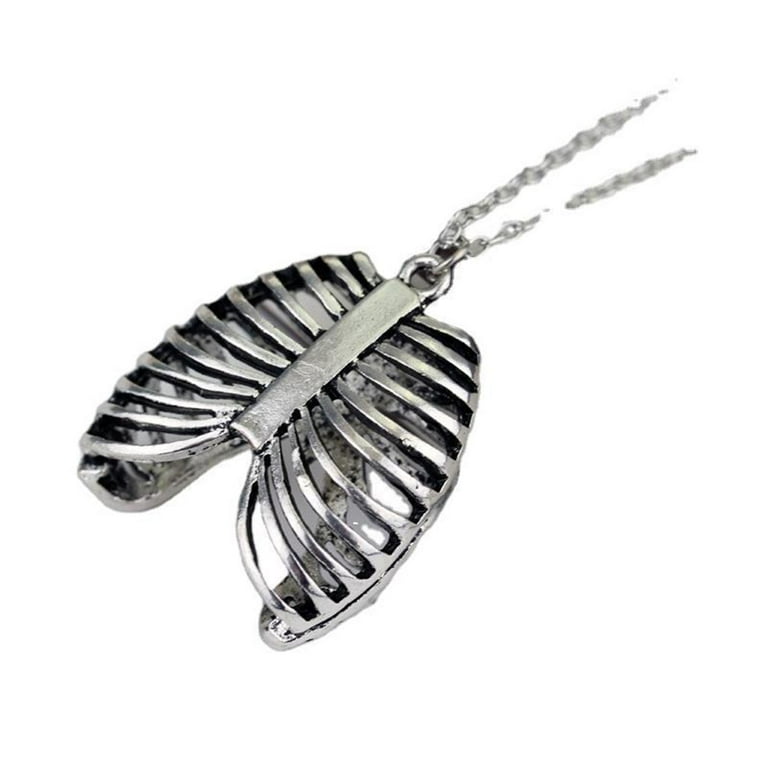The image depicts a silver necklace, featuring a pendant shaped like a human rib cage. The rib cage pendant is crafted from a chrome or silver-colored metal and includes 11 bars or openings, mimicking the structure of a rib cage, complete with a breastbone. The pendant hangs on a fine silver chain, which is visible in the photo. The background of the image is plain white, though it appears to have been edited to remove the original background, resulting in some choppy edges. Shadows are present, suggesting the piece might not be of the highest craftsmanship. The image seems tailored for online marketplaces like Etsy or eBay, possibly targeting niche buyers such as medical professionals.